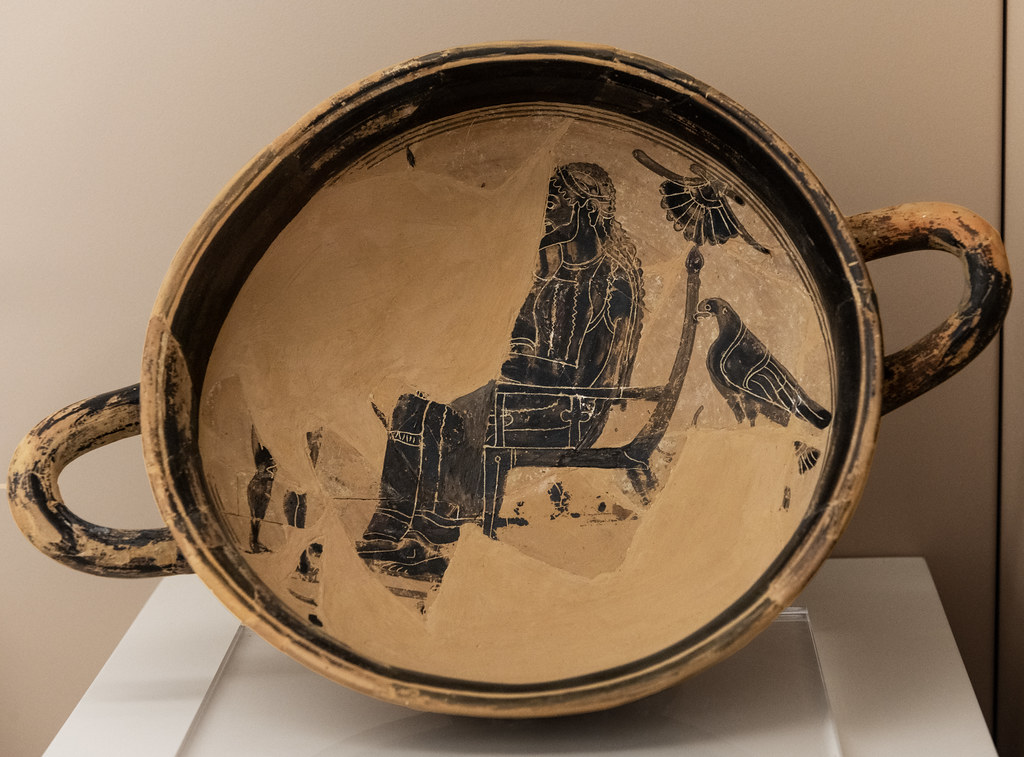This color photograph depicts an artifact, potentially Native American pottery, on display. The pottery piece is a jug or plate with a distinctive cream to light brown, almost orangey-tan coloration. Positioned on a white square exhibition pedestal, the artifact is turned sideways to showcase its intricate design. The jug features two splotchily black-painted handles with orange-yellow blotches. The inner lining of the jug is black, housing a hand-drawn image in black ink. This image depicts a man sitting in profile, with one or possibly two birds to his right. Notably, parts of this image appear to have been scratched or worn away over time. The background wall against which the artifact is displayed is a tan-cream color, complementing the earthy tones of the pottery.